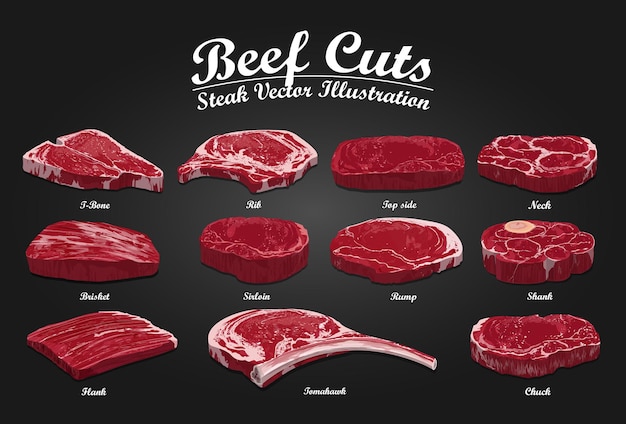This animated image presents a detailed overview of various beef cuts, organized into three horizontal rows against a dark gray background. There are a total of 11 beef cuts depicted. The bottom row features three cuts: a square-shaped cut on the far left, a circular cut with a bone in the middle, and an oval-shaped cut on the right. 

In the middle row, starting from the right, there is a uniquely shaped cut with a couple of circular edges, and next to it on the left, a flat, circular cut labeled "Ramp." Further left, there's a thick, circular cut labeled "Shlein," and the leftmost cut in this row is labeled "Brisket."

The top row showcases four cuts, starting from the left: "T-Bone," followed by "Rib," then "Top Side," and the rightmost cut labeled "Neck." 

Above all these cuts, the title "Beef Cuts, Steak Vector Illustration" is written in white cursive text, providing a concise description of the image's content.